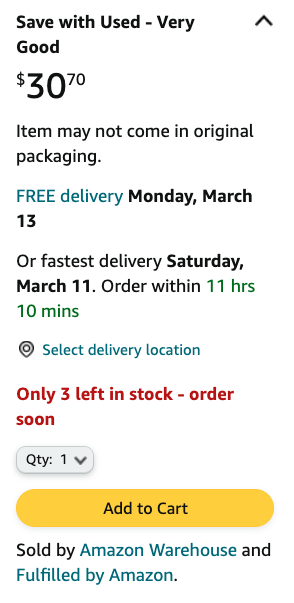**Screenshot Description: Online Shopping Interface**

The image is a screenshot of an online shopping interface with a white background. In the top right corner, there is a black, upward-pointing greater-than sign. The text on the screen is primarily black, with key elements highlighted in blue, gray, red, and yellow.

On the left-hand side, bolded text reads, "**Save with Used - Very Good**." Below that, the price is listed as "**$30.70**." Following the price, it states, "**Item may not come in original packaging**."

In a blue font, the word "**FREE**" (in all capitals) appears, followed by "**delivery**" in black. The estimated delivery date is then provided as "**Monday, March 13**." A small space separates this from the next line.

Further down, the text indicates that expedited shipping is available with the message, "**Or fastest delivery Saturday, March 11. Order within**," continuing in gray text with, "**11 hours 10 minutes.**" Adjacent to this line is a location icon and the option in blue to "**Select delivery location**."

Following another small space, the text warns in red, "**Only 3 left in stock - order soon**."

Below, there is a small gray tab containing the text "**QTY: 1**" with a downward-pointing greater-than sign, signifying a quantity selector.

A yellow-orange tab spans the width of the section, with centered black text stating, "**Add to Cart**" (with "Add" and "Cart" capitalized).

Underneath this button, the text reads in black, "**Sold by**," followed by the seller, "**Amazon Warehouse**" in blue. Finally, the fulfillment information is stated in blue as "**Fulfilled by Amazon.**"